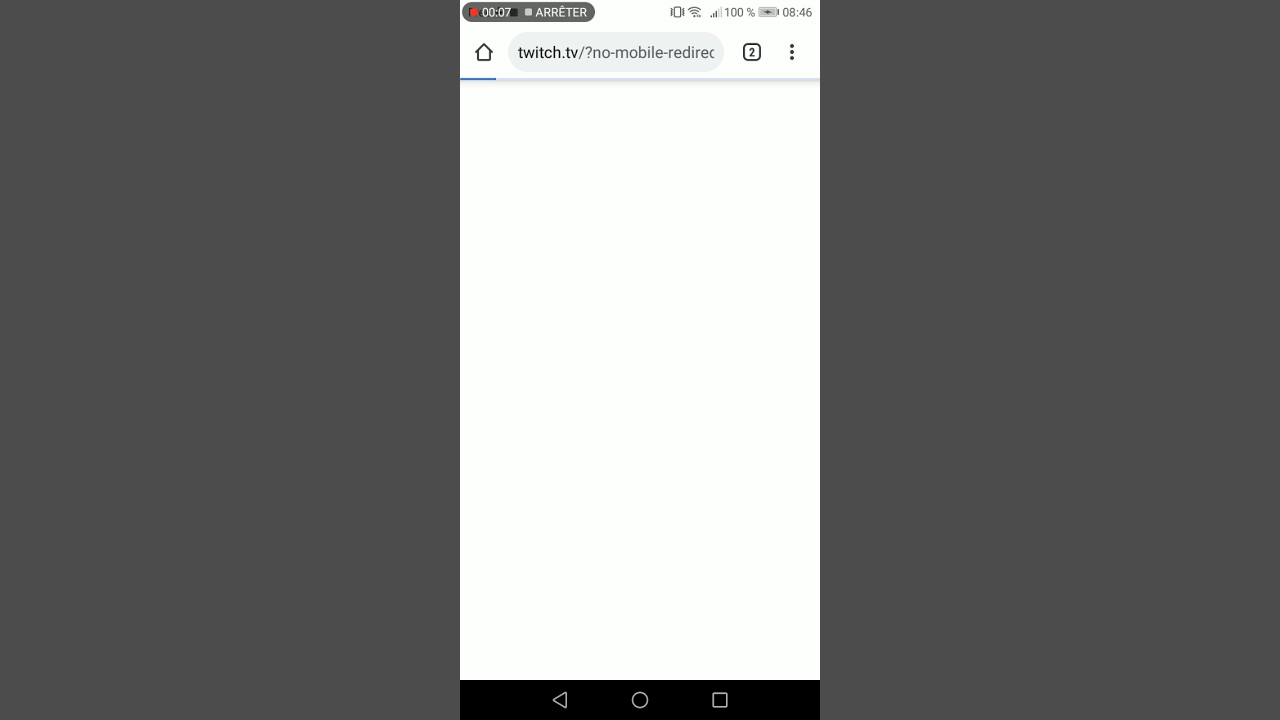A screenshot displays a partially loaded browser screen where a user has typed into the search bar on Twitch TV, seeking information or a specific channel. The screen shows a redirect happening, with the search result failing to load fully. The progress bar at the top indicates minimal progress, hinting at a stalled or frozen state. The screen remains largely blank, except for the markers displaying "0.07 seconds" and "ARRETER" in the top left corner, signaling the duration before the attempt stopped. On the right, standard status icons are visible: full Wi-Fi signal, cell signal, and a fully charged battery at 100%. The time on the device reads 8:46. Additionally, two browser tabs are open, as indicated by the tab count next to the search bar.